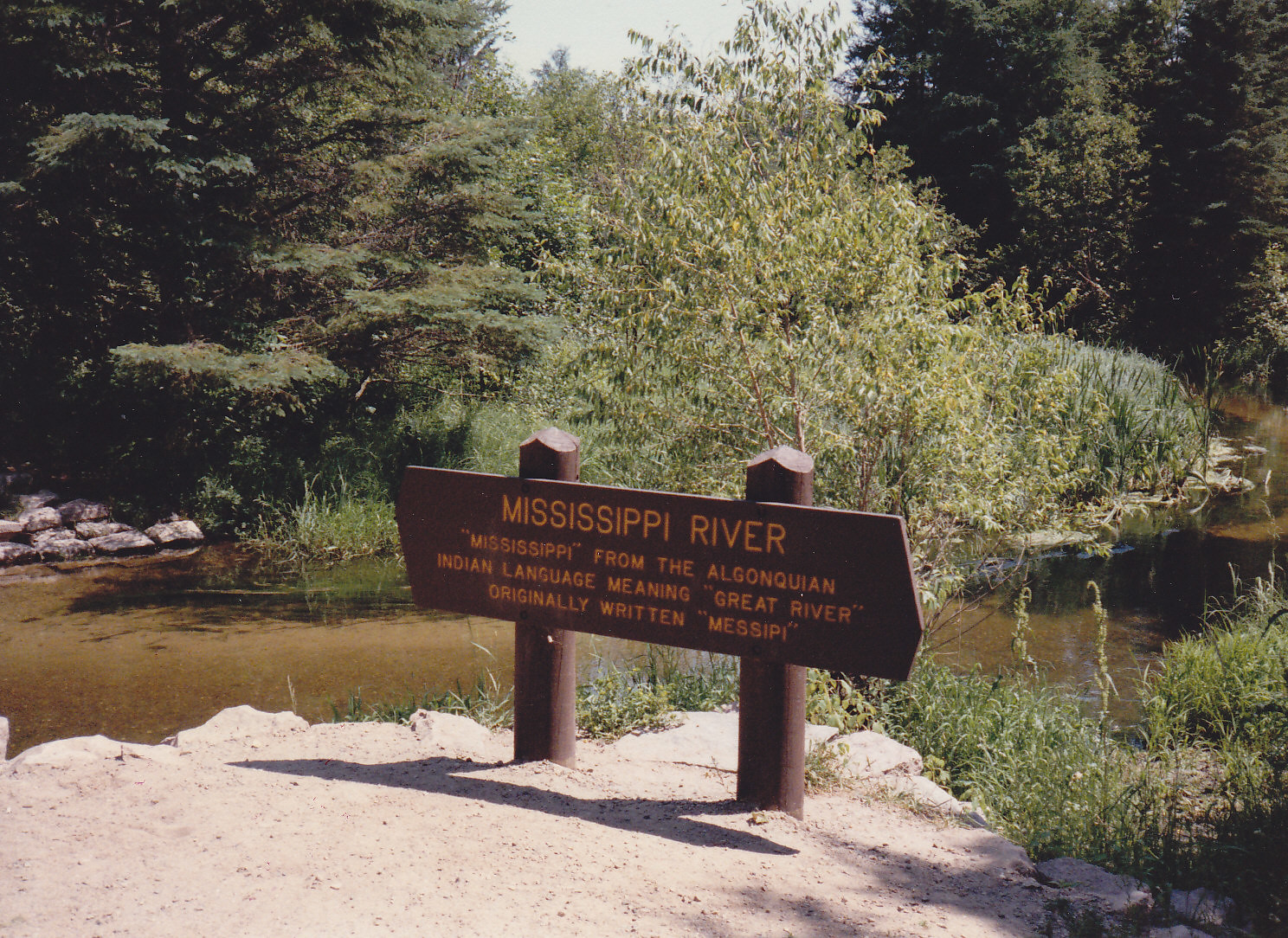In this outdoor image, a wooden sign bearing the label "Mississippi River" stands firmly affixed to two dark brown cylindrical poles, each about three to four feet high. Positioned on a sandy, light gray soil that resembles barren dirt, the sign is placed slightly to the bottom left of the center. The ground beneath it is devoid of plants or vegetation, giving it a stark appearance. The sign itself is wider than it is tall, adorned in an orange-colored font, stating: "Mississippi River. Mississippi from the Algonquian Indian language meaning Great River, originally written Mississippi."

Behind this sign lies a shallow body of greenish-brown water, almost appearing as a small brook or stream. Extending further into the background, tall, lush green trees form a dense canopy that obscures much of the sky, though patches of pale gray sky can still be glimpsed. The sun's early afternoon light casts distinct shadows of the sign and poles onto the sandy surface below. The overall tone of the image suggests an aged photograph, with a slight yellow hue that adds a timeless quality to the scene.